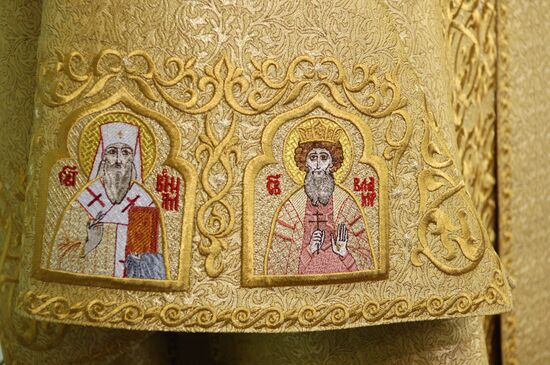This highly detailed and ornate image appears to be an intricate piece of ecclesiastical embroidery possibly from a Catholic or Orthodox Christian tradition, stitched onto a richly golden fabric, perhaps a robe or another form of sacred garment. It depicts two distinguished figures, each adorned with symbolic clothing and accessories.

On the left, a priestly figure with a long white beard is prominently featured. He is wearing a white hat and a white garb adorned with red crosses on the shoulders, along with an orangey-red sash draped over one shoulder. His hand is raised, with fingers pointed in a gesture of blessing, a golden sunbeam halo illuminating his head, and intricate red symbols stitched around him.

To his right, a second figure, possibly a king, is depicted with brown, curly, afro-like hair, a gray beard, and a golden crown. Clad in elaborate robes, he is holding a cross aloft, his other hand raised in a gesture. Both figures are surrounded by ornate stitching and red lettering, enhancing the detailed craftsmanship of the piece. The artwork is likely zoomed in, focusing on just these two significant personalities, highlighting the rich tradition and reverence in the intricate needlework.